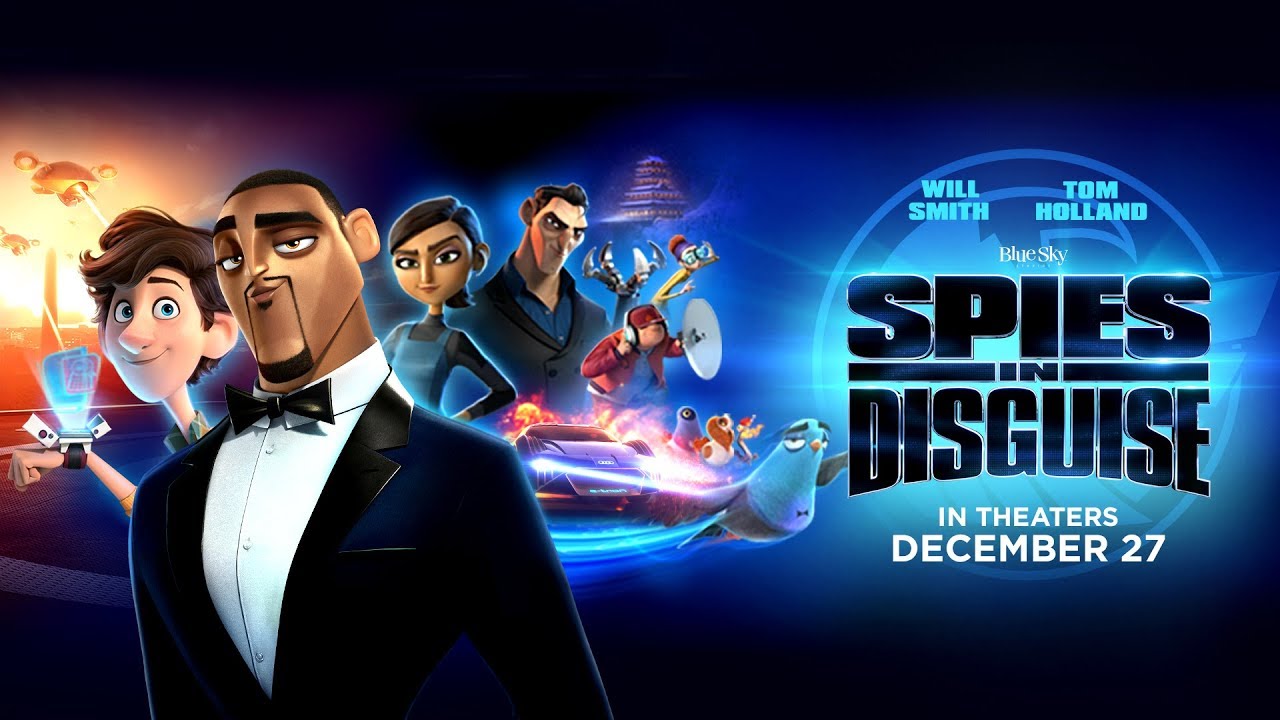The advertisement is for an upcoming animated film titled "Spies in Disguise." On the far right, the film's title and logo are displayed in bold black letters, surrounded by vibrant neon blue in a circular pattern. Beneath the title, it reads "In theaters December 27th" in white letters. The banner prominently features renderings of the main characters, voiced by Will Smith and Tom Holland. 

On the left side, a cartoonish depiction showcases Will Smith as an African-American gentleman with a goatee, dressed sharply in a tuxedo, with an angular animated face. Beside him stands Tom Holland’s character, a younger white boy holding up a watch, from which an image is projected. The background also includes other cartoon characters: a woman of ambiguous race with short dark hair and medium dark skin, standing confidently with her hands on her hips, exuding a sassy demeanor; behind her, a man who appears to be a villain, dressed in an open-collar suit with a strong face and dark hair. Additional elements like claws, birds, a car, and possibly a spaceship add to the action-packed feel of the advertisement. The entire background has a predominantly blue theme, with black bars at the top and bottom. This visually dynamic banner effectively promotes the film "Spies in Disguise," generating excitement for its release on December 27th.